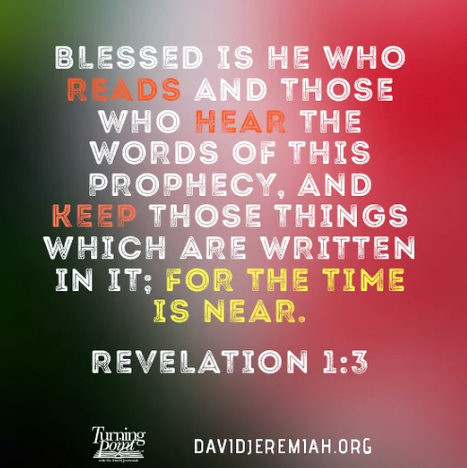The image showcases a Bible verse placed prominently against a gradient background. The gradient transitions from black with dark green at the top on the left side, to a more white center, and moves into shades of red, pink, and gray on the right. At the center of the image, various lines of text are displayed in different colors. It reads: "Blessed is he who reads" (in white), "and those who" (in white), "hear" (in orange), "the words of this prophecy" (in white), "and keep" (in orange), "those things which are written in it" (in white), "for the time is near" (in yellow). This Bible verse is from Revelation 1:3. Beneath the verse, in the bottom center of the image, is the website URL "davidjeremiah.org." To the left of the URL, there is a logo that reads "Turning Point" in white font above a side view graphic rendition of a book.